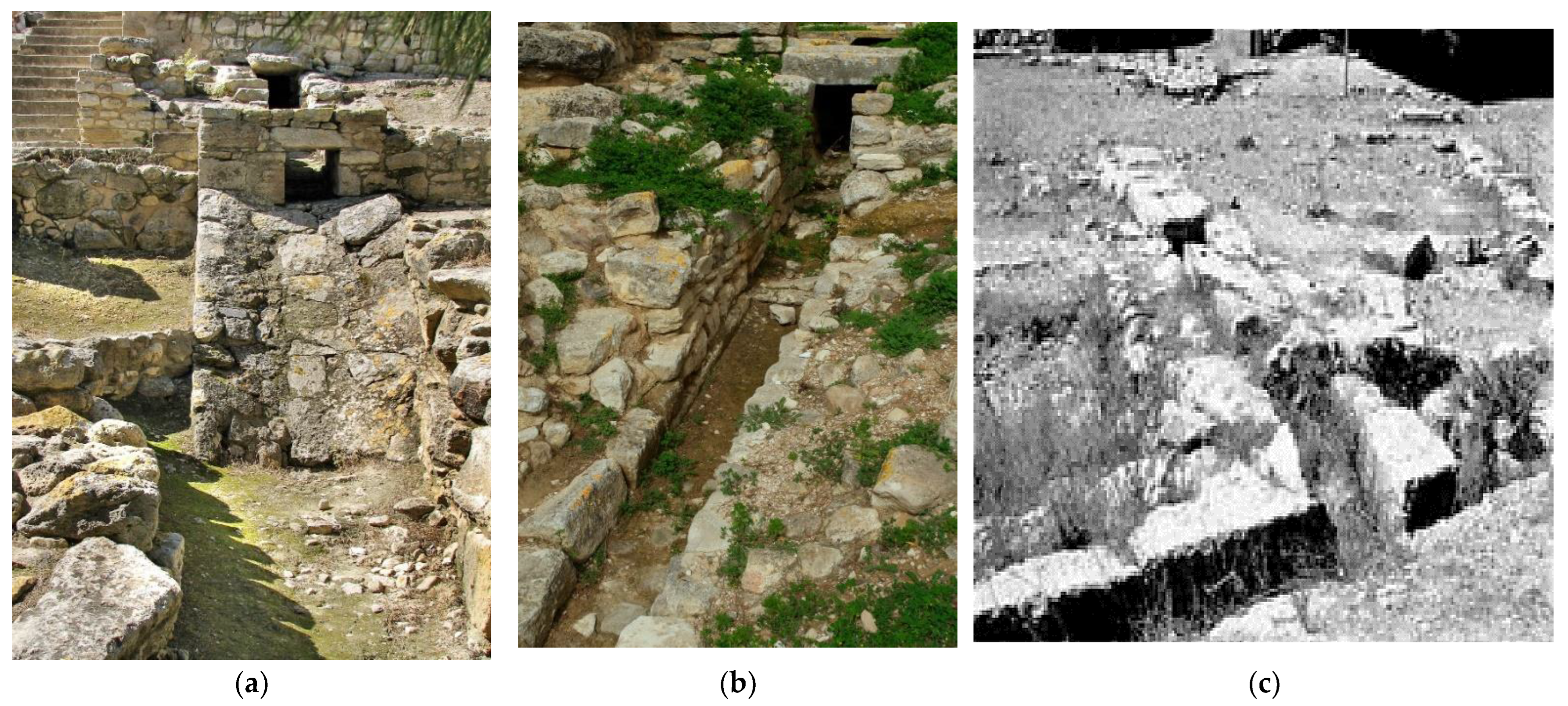This horizontal rectangular frame features three side-by-side photographs of archaeological sites, labeled A, B, and C. 

- **Image A** (left) is a daylight color photo showcasing the ruins of an ancient stone structure. Tall standing walls form various right-angled patterns, with some sections appearing damaged and irregular on top. The background reveals a higher wall with steps leading upward to the left, possibly into the remains of an internal structure. The ruins sit on what seems to be a grassy or mossy field, highlighting the site's weathered but majestic presence.

- **Image B** (center) is another daylight color image, depicting an intricate maze of uncovered passages and foundation walls amidst rubble. The stone floors are partially covered with patches of moss. In the top right corner, a dark doorway punctuates the stone formations, hinting at an entrance or corridor within the ruins.

- **Image C** (right) is a black and white photograph that, though blurry and high-contrast, still conveys an atmosphere of ancient desolation. It shows similar passageways between stone walls but with indistinct details. The photograph appears to be taken under low light or nighttime conditions, making specific elements harder to discern.

Together, these images provide a comprehensive look at the archaeological site, capturing both the detailed masonry of individual structures and the overall layout of the area.